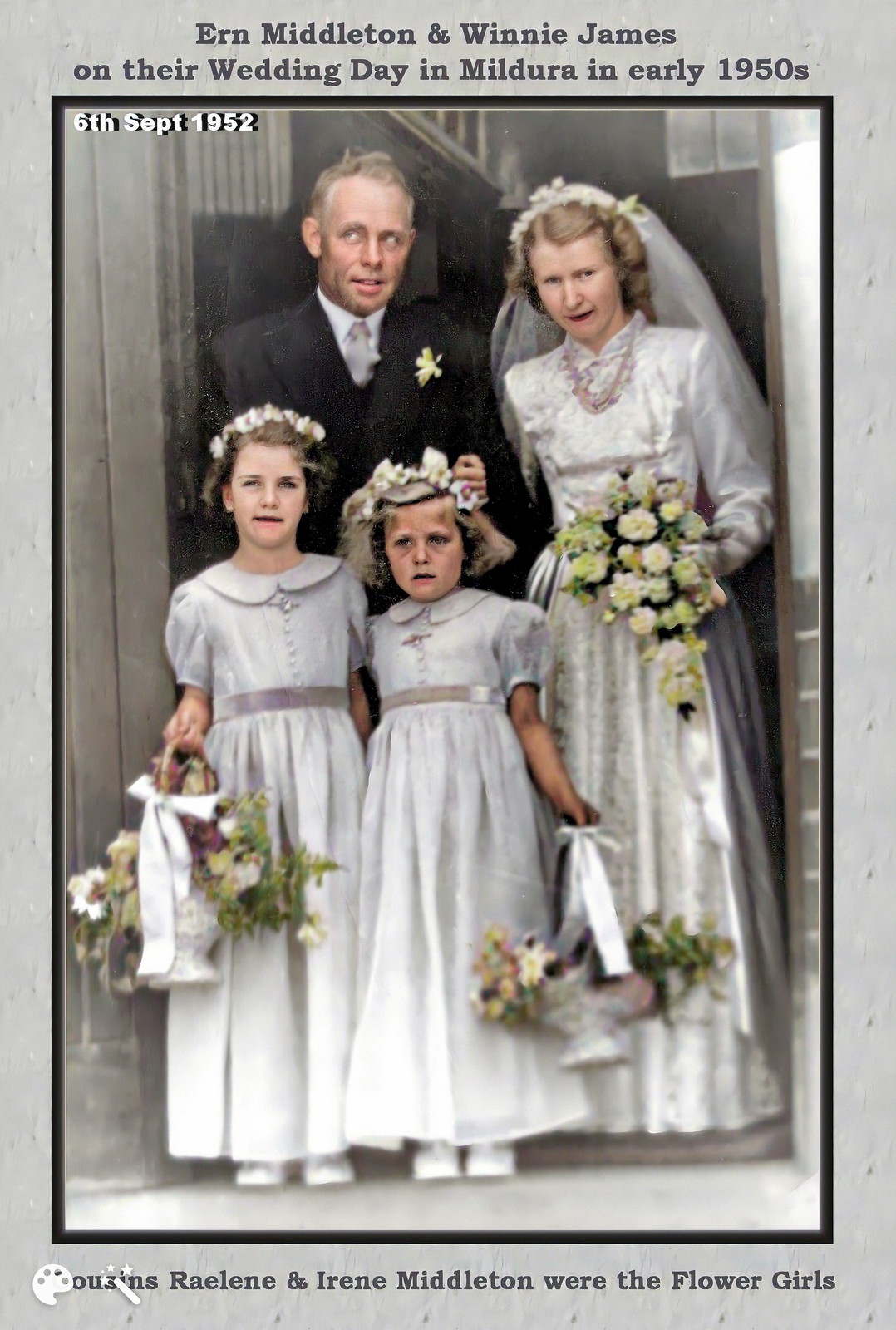The image is an old, color photograph framed with a gray border, featuring a wedding scene from Mildura on the 6th of September, 1952. The image depicts Erne Middleton and Winnie James on their wedding day. Winnie, the bride, stands in a white wedding gown, holding a bouquet of white and green flowers that appear to have been color-enhanced. She wears a pink necklace, a white headdress, and has blonde hair. Beside her is Erne, dressed in a black suit, gray tie, and white collared shirt. His hair looks short and gray. In front of them are two young flower girls, Raylene and Irene Middleton, cousins of the couple. The flower girls are also in white dresses with beige sashes and carrying flower baskets. The detailed attire and the serene doorway setting frame this nostalgic moment perfectly. The writing on the gray border of the image provides a timeless caption, documenting this beautiful occasion.